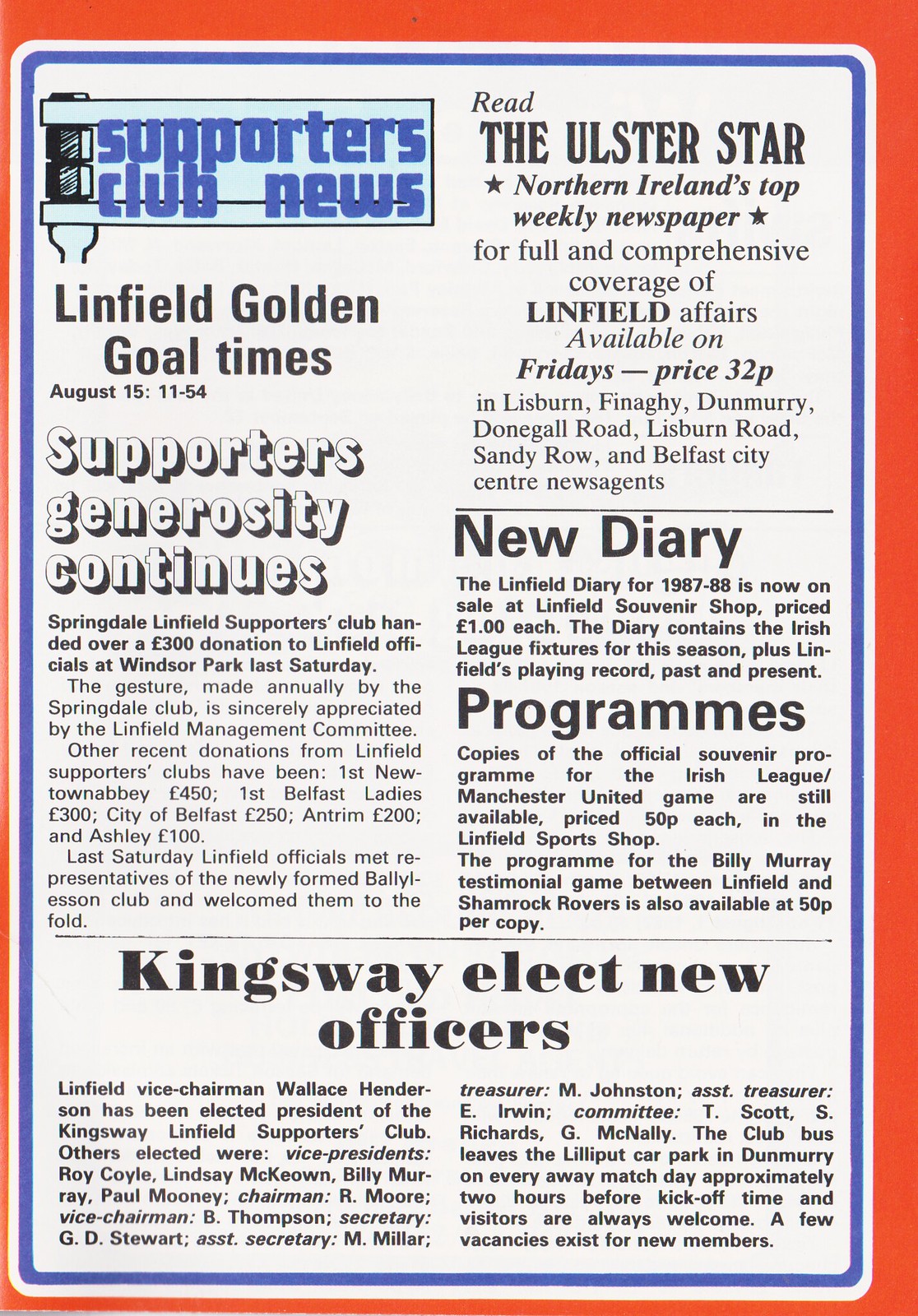The image depicts a detailed clipping, possibly from a newspaper or a magazine, with a thin dark orange outline framing it and a central rectangle featuring a blue border. In the upper left corner, set against a blue background, the text reads "Supporters Club News." Beneath, it states "Linfield Golden Goal Times, August 15, 11:54." The main headline, "Supporters' Generosity Continues," headlines an article consisting of three to four paragraphs. 

On the right side, another column begins with "Read the Ulster Star, Northern Ireland's top weekly newspaper for full and comprehensive coverage of Linfield affairs. Available on Fridays, price 32p." A note mentioning availability at Bisban, Majorie, Don go Rodent, Road Sandy Road, and Built This City Center News Agents follows. 

A black bar separates this column from the subsequent sections labeled "New Diaries" and "Programs." At the bottom, a section titled "Kingsway Elect New Officers" contains two additional paragraphs of text. The overall color scheme features a primarily white background with black and blue text, enhanced by red and blue highlights. The layout and content suggest a program or pamphlet dedicated to sports club news.